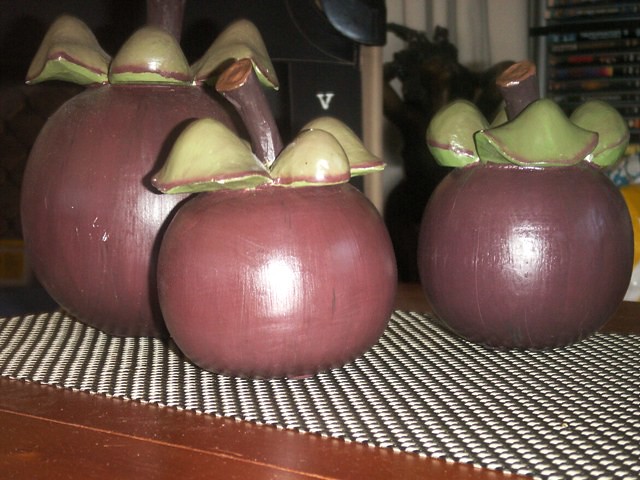In the image, we see a close-up of three decorative apple-shaped ornaments placed on a woven black-and-white placemat. The ornaments are intricately crafted, likely from wood or ceramic, and exhibit a reddish-purplish hue with visible wood grain beneath the paint, making them appear somewhat stylized. They are topped with greenish leaves and substantial, brownish-purple stems. The arrangement includes one larger apple in the background and two smaller ones in the foreground, each varying slightly in size. The placemat sits on a dark brown wooden table, hinting at age through its modest wear.

The scene appears to be set in a home, indicated by the light gray window curtain and various household objects and DVDs visible on shelves in the blurred background. The photograph itself is amateur and landscape-oriented, with colors suggesting it was taken some years ago, adding to the nostalgic ambiance. Overall, the quirky, oversized apples exude a charming, rustic appeal in this cozy domestic setting.